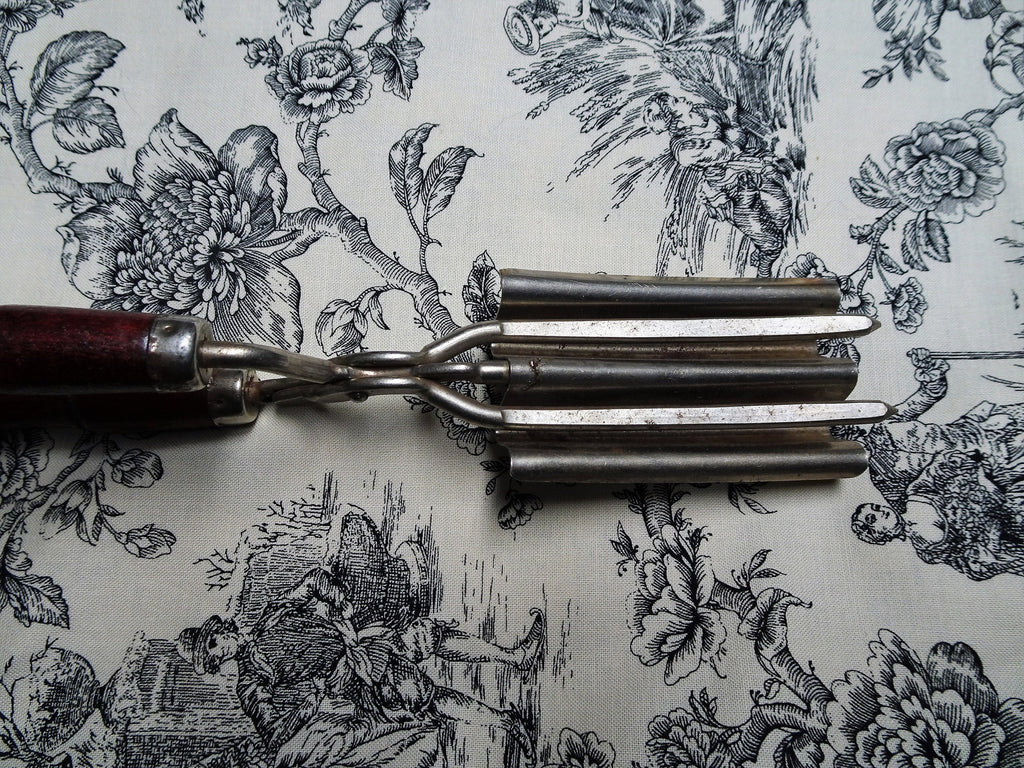This photograph features an old-time stirring tool, characterized by its silver metal construction and wooden handles that are reddish-brown in color. The tool has multiple prongs or blades at the end, which could be for mixing food or other substances. The central focus of the image is this antique tool, which sits horizontally against a striking black-and-white background. The background appears to be wallpaper or fabric adorned with detailed designs, including a man dressed in old-fashioned attire—knee-length breeches, curved shoes, leggings, a wrap tie around his waist, a long-sleeved shirt, and a hat. Surrounding this central figure are various elements of nature, such as trees and flowers, enhancing the overall vintage feel of the scene. The elaborate backdrop sets an evocative tone, reminiscent of the old country.